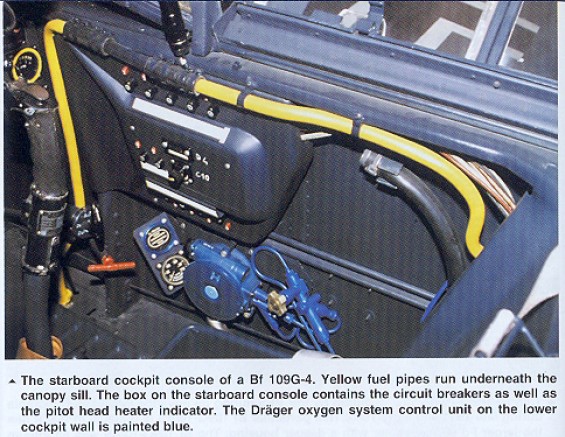The image is a square photograph capturing the intricate interior of a BF 109 G-4 cockpit. Dominating the scene, the starboard console features prominently with a box containing circuit breakers and the pitot head heat indicator. Visible in the lower section of the cockpit wall is the blue-painted Draeger oxygen system control unit. The backdrop includes a light blue panel stretching diagonally from the upper left to the right side of the image. Strikingly vibrant yellow fuel pipes traverse horizontally beneath the canopy sill, with some extending vertically. Additional cockpit details include various gears, levers, wires, and an orange handle, all set against a black floorboard. The overall color palette of the cockpit is a mix of light blue, dark blue, and yellow, giving it a distinct, albeit somewhat aged, appearance. The textual description at the bottom against the light blue background, presented in left-aligned black text, provides a functional overview of these features for easier understanding.